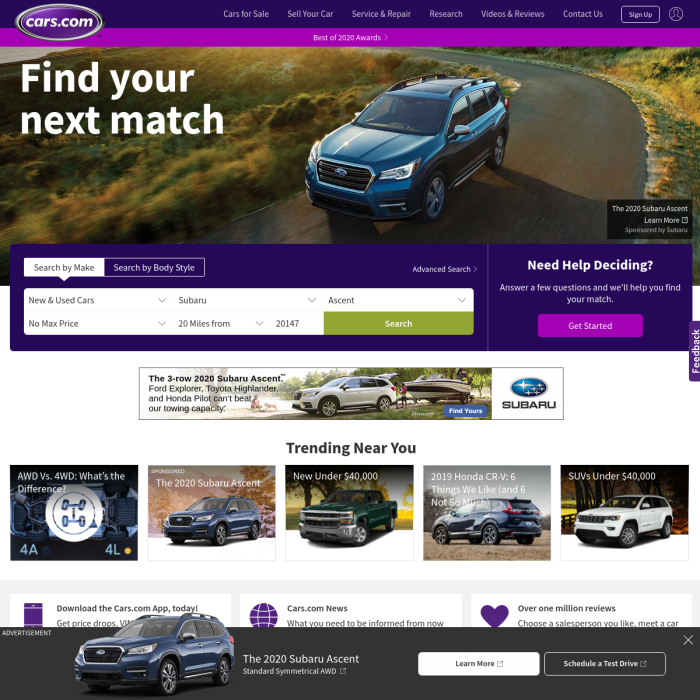This screenshot showcases the homepage of cars.com, a website dedicated to car sales, with a distinct purple color scheme. The layout features a dark purple header at the top, followed by a lighter purple header beneath it. Central to the design is a landscape-oriented image of an SUV driving towards the camera on a rural road flanked by lush, green hills. Prominently displayed at the top is an oval logo in purple with a silver border that reads "cars.com" in white text.

Above the SUV image, a series of clickable text links provide navigation across the website. Directly below the image, set within a dark purple box, are search filtering options with drop-down menus to select car make, price range, mileage, and condition (new or used), enabling users to refine their search criteria. At the bottom of the screen, a pop-up ad appears, requiring users to click "Next" to dismiss it and continue browsing. This functional and visually appealing design aims to streamline the car search process for users.